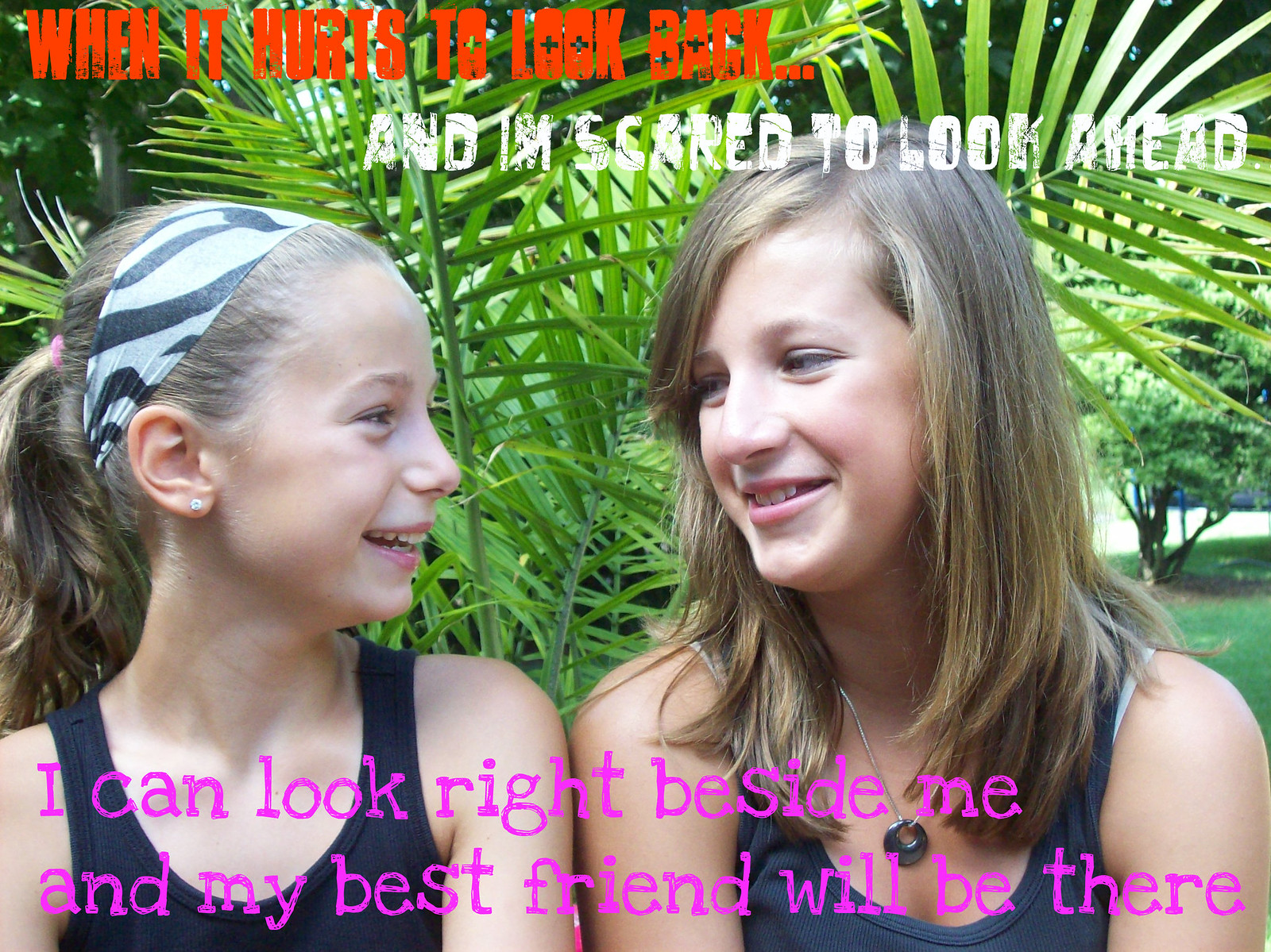The advertising poster features two young girls sitting close together and looking at each other with bright smiles. The background showcases thin-leaved palm plants, giving a tropical atmosphere. At the top left corner, in red lettering, it reads: "When it hurts to look back," and below that, in white letters: "And I'm scared to look ahead." At the bottom, in purple lettering, it states: "I can look right beside me and my best friend will be there." Both girls are approximately 13 or 14 years old. The girl on the left has her hair pulled back in a ponytail, secured by a zebra-patterned hairband, along with a small earring. She is wearing a black, narrow-sleeved cami top and looking happily at her friend. The girl on the right, slightly taller, has long blonde hair cascading over her shoulders. She is also smiling warmly at her friend and wears a sleeveless blouse similar to the other girl's. Around her neck is a silver necklace with a disc pendant that has a hole through which the chain passes. The overall mood captured in the poster is one of close friendship and mutual support.